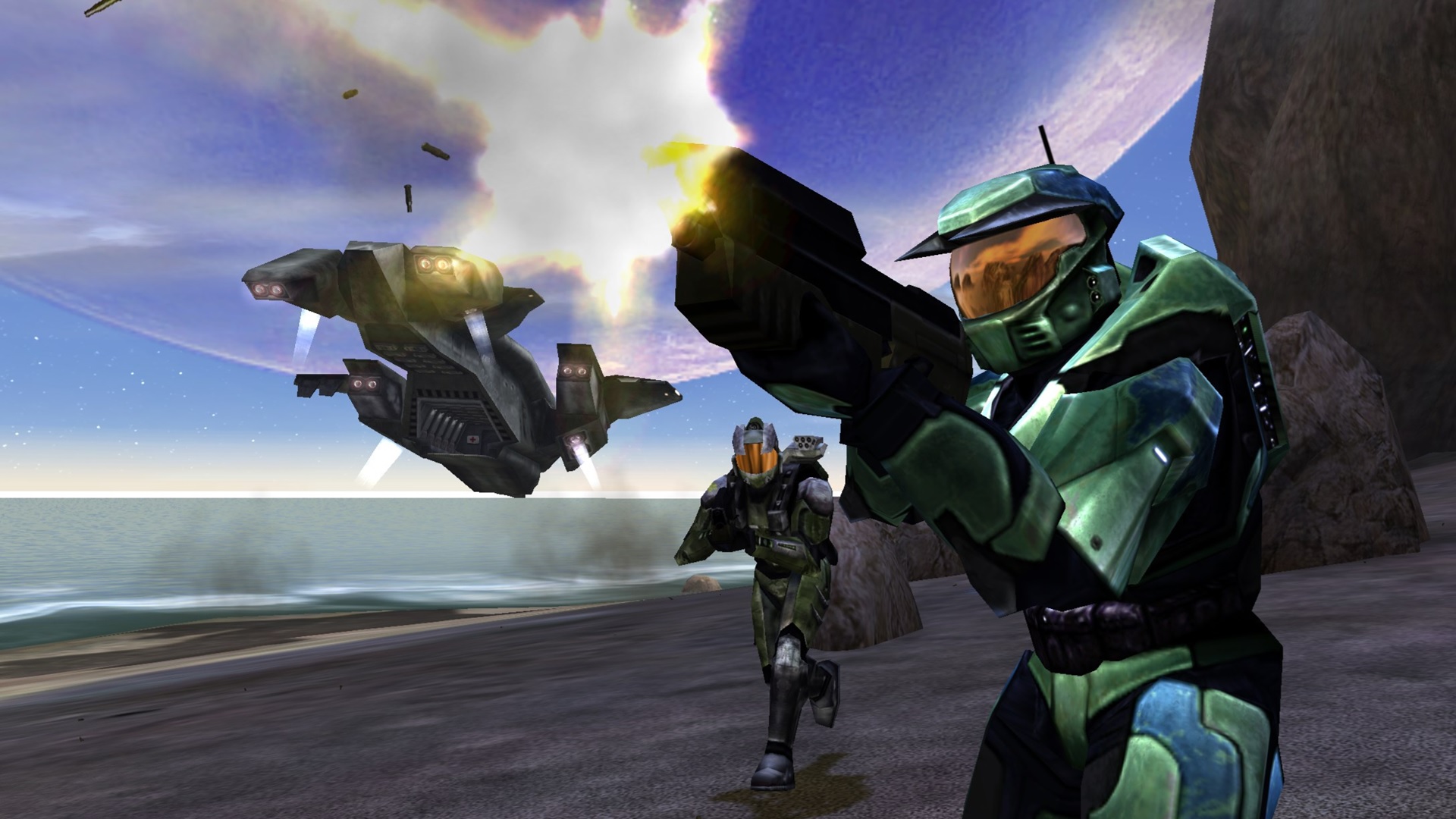In the image, which appears to be a scene from the video game Halo or a similar futuristic battle setting, a dramatic space battlefield unfolds against a striking celestial backdrop. Central to the scene is a man clad in a green mech suit with blue accents and black portions, featuring a reflective tan visor. This soldier is firing a large gun that releases a burst of bright yellow energy accompanied by white smoke and bullet fragments. The yellow burst then narrows into a string trailing from the weapon.

To his left, a fellow warrior in a similar, though more gray and silver, mechanized suit runs forward, holding a gun but yet to fire. Both soldiers appear on a gray, tarmac-like surface, suggesting a combat zone. They stand before massive rock formations jutting into the sky on the right.

The background is rich with details: A green-hued ocean lies beneath a blue sky, and farther in the distance, a transport aircraft with two wings is seen ascending or possibly in a downward trajectory, trailing smoke as if damaged. Above this, a gigantic moon with shades of purple, white, and blue dominates the sky, adding to the otherworldly atmosphere of the scene. This barren, extraterrestrial landscape provides a stark, dramatic setting for the unfolding battle.